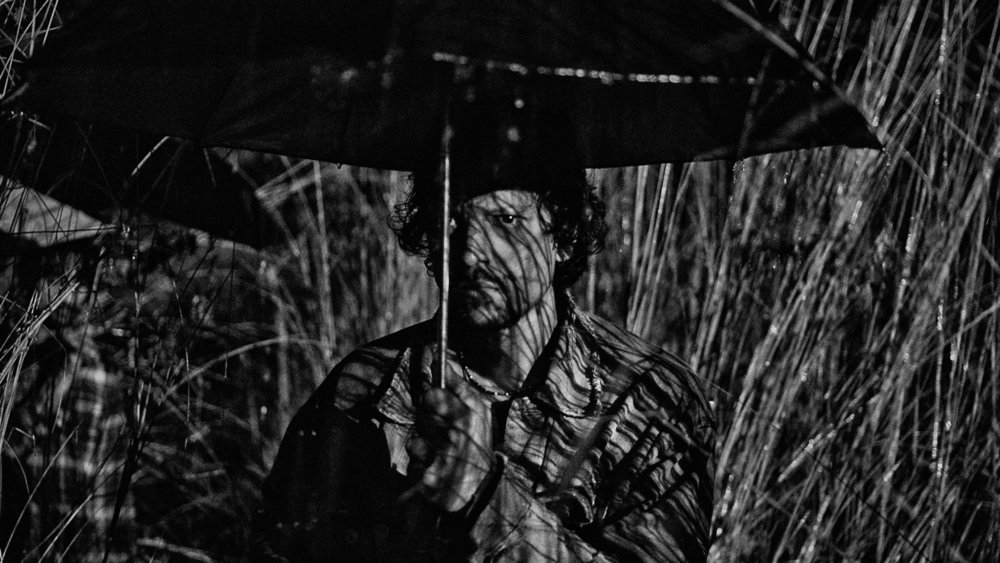The image is a screenshot of a black-and-white movie scene displaying a man standing amidst tall, pond-side grasses. The man’s stern, determined, and somewhat sinister expression is accentuated by shadows cast by the long grass onto his face and upper body, giving the appearance of dark lines streaking across his features and jacket. He's holding a dark umbrella close to his chest, which offers some protection from the rain drizzling down onto his medium-length, slightly wet, and disheveled hair. His attire includes what appears to be a collared t-shirt or a raincoat, and the photograph captures everything from his chest up. The scene is dark, and the contrast of shadows and light heightens the dramatic atmosphere surrounding the man.